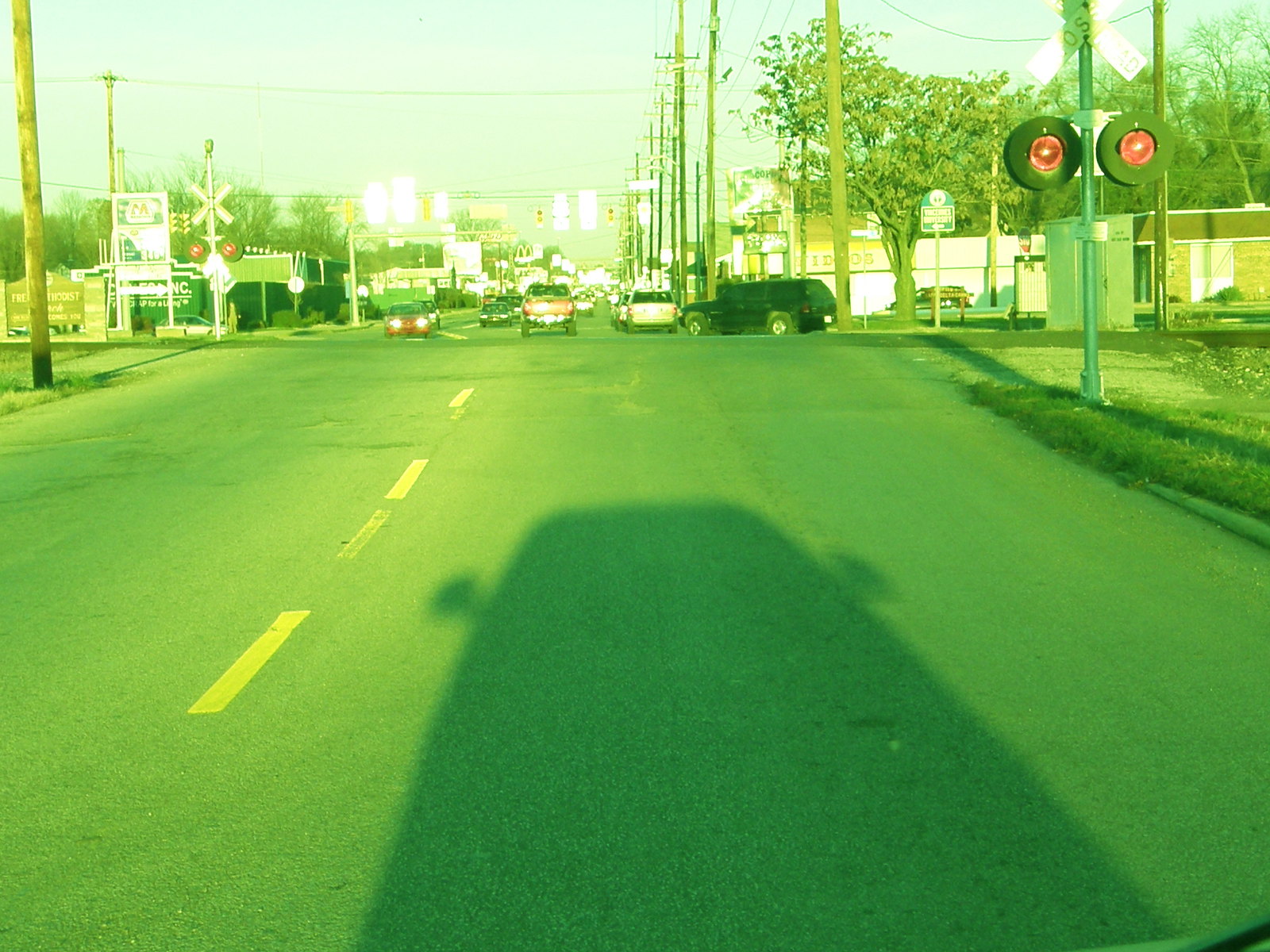The image showcases a serene suburban town beneath a partly cloudy sky, where patches of blue peek through scattered white clouds. At the bottom of the image, a green-hued road runs across, casting the shadow of an unseen vehicle. On the right side, a set of railroad tracks extends into the distance, framed by lush green scenery. The image overall has a green tint, adding to its tranquil, nature-rich atmosphere. This location appears familiar, evoking a sense of familiarity and calm.